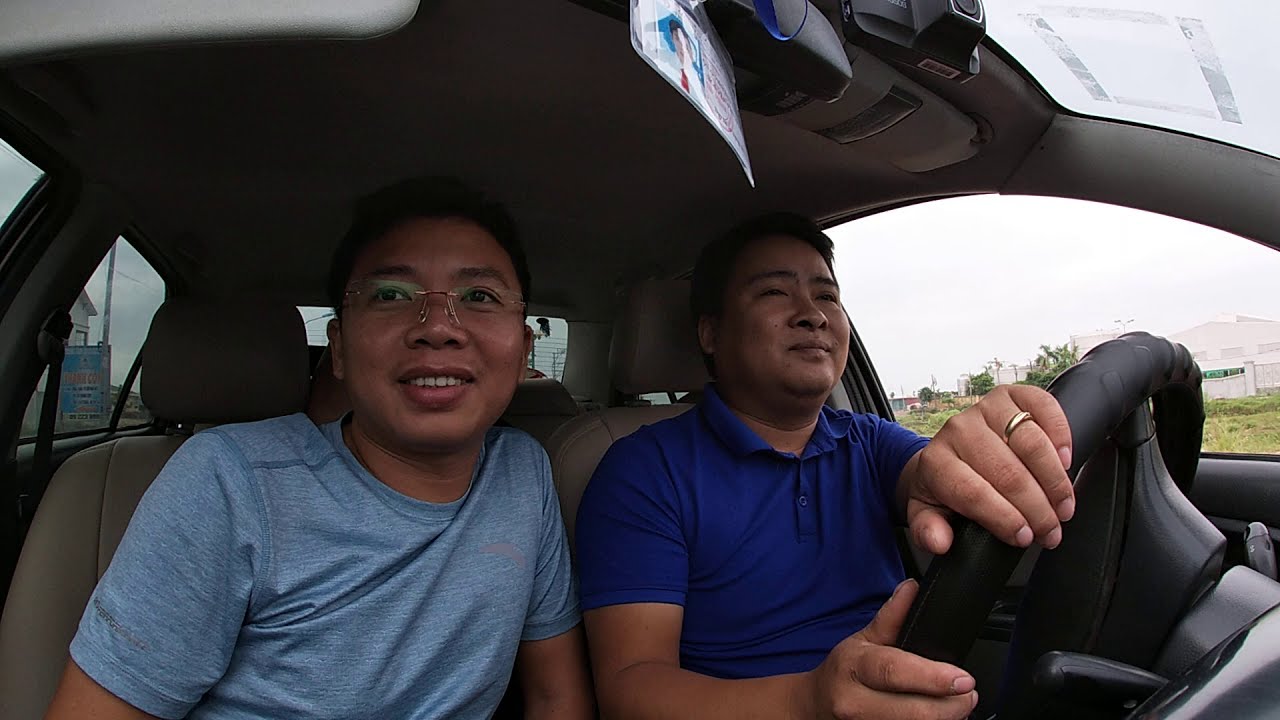This daytime photograph, taken from a dashboard camera, captures two men of Asian descent sitting in the front seats of a car, set against an urban backdrop with visible trees, greenery, and buildings. The man in the driver's seat, positioned on the right, is clad in a royal blue polo shirt and wears a golden wedding band on his left hand, which is firmly gripping the chunky black steering wheel as he appears to be making a right turn. He has short dark hair and a closed mouth. To his left, in the passenger seat, is a younger-looking individual sporting a light blue t-shirt and light-framed glasses. This passenger has short dark hair as well, and his mouth is slightly open, revealing his teeth slightly. Above them, the rearview mirror is visible, along with another camera and a worker's badge hanging from it. The overall scene is well-lit, suggesting it was captured in bright daylight or under a white overcast sky. The interior of the car features light gray seats, and outside the driver’s side window, you can see a mix of green ground and gray buildings, indicating an urban setting.